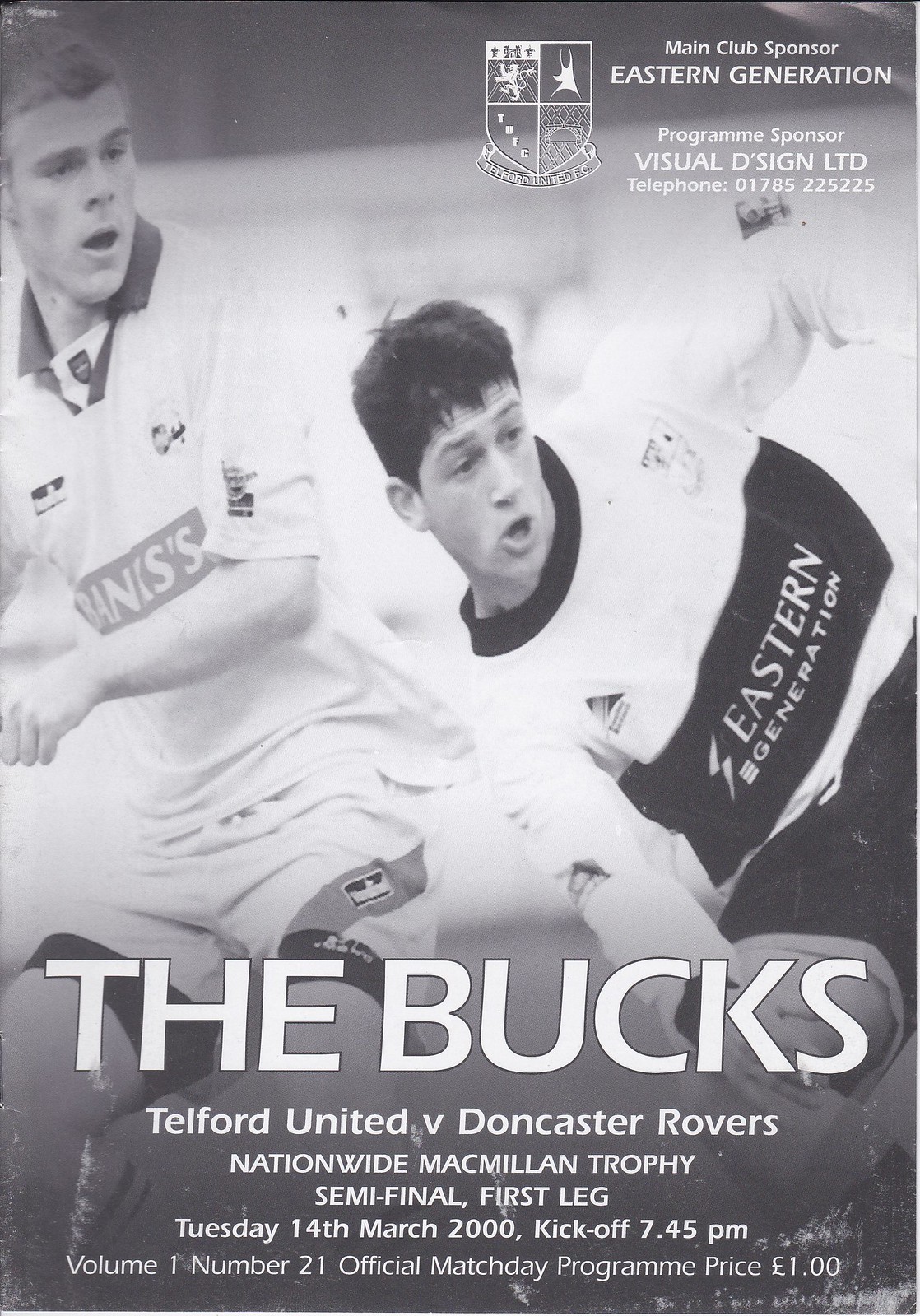The image features the front page of a scanned, black and white soccer match program. Dominating the page, a dynamic photograph captures two Caucasian male soccer players in action, battling for the ball. One player wears a uniform branded with "Eastern Generation," while the other sports a different sponsor, though the text is unclear. 

In the upper right corner, the text reads "Main Club Sponsor: Eastern Generation," and beneath a shield symbol, it states "Program Sponsor: Visual Design LTD," followed by a phone number, "01785-225-225." The bottom of the page prominently displays "The Bucks" in uppercase letters, alongside essential match details: "Telford United vs. Doncaster Rovers, Nationwide Macmillan Trophy, Semi-Final, First Leg, Tuesday 14th March 2000, Kickoff 7:45 PM." The program is identified as Volume 1, Number 21, and is marked "Official Match Day Program" with a price tag of "1 British Pound."